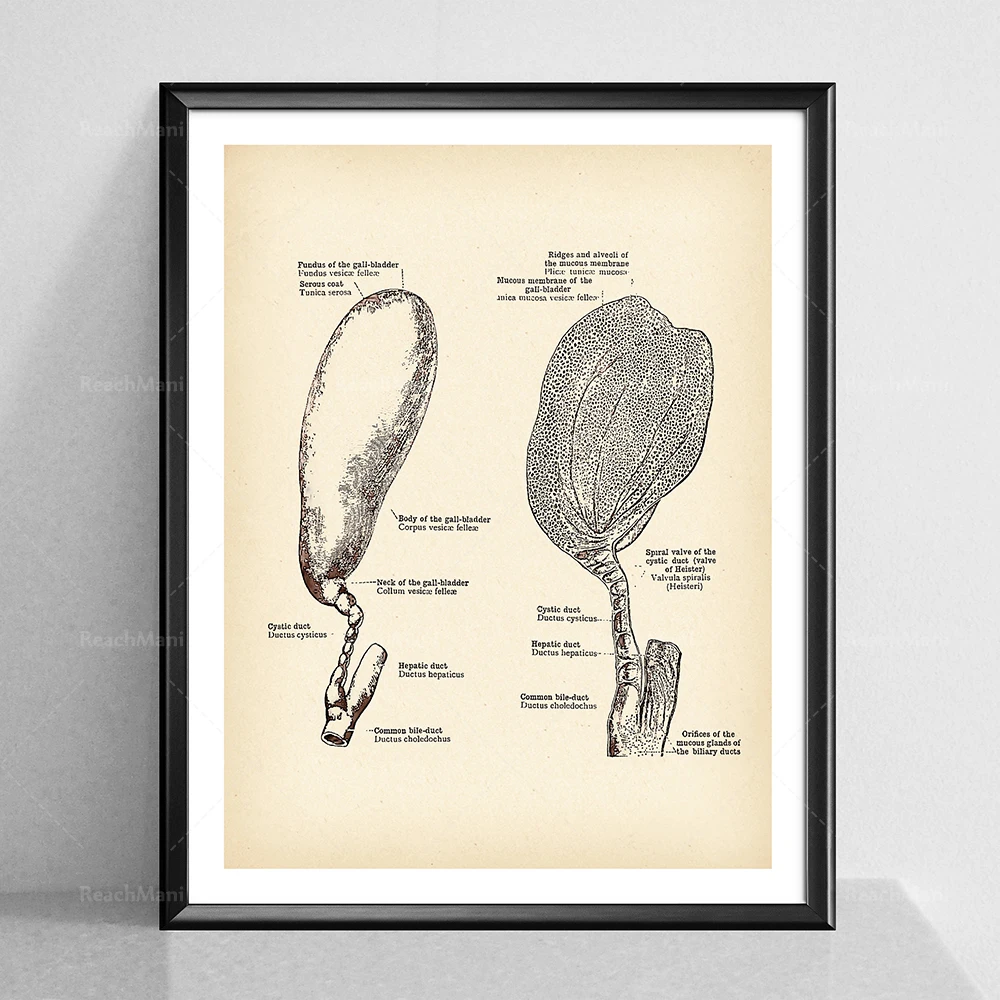The image features a framed diagram of a gallbladder, prominently stamped with the watermark "Reach Mini." The frame is either wooden or metallic in black, with a white inner border, encasing a weathered light brown diagram. The background wall is white, creating a stark contrast. The gallbladder is depicted in two separate illustrations. The left illustration resembles an oblong shape, akin to a potato or eggplant, with a stem-like extension, and is bordered in black but remains unfilled with shading. The right illustration is a bulbous shape with extensive shading and dotted details, possibly indicating gallstones or inflammation. Both diagrams include detailed labels such as "ridges and alveoli of the mucous membrane of the gallbladder," "spiral valve of the cystic duct," "fundus of the gallbladder," "body of the gallbladder," "neck of the gallbladder," "cystic duct," "hepatic duct," and "common bile duct," with arrows pointing to these specific parts. The overall image is in black and white, giving it an antique, scientific illustration feel.